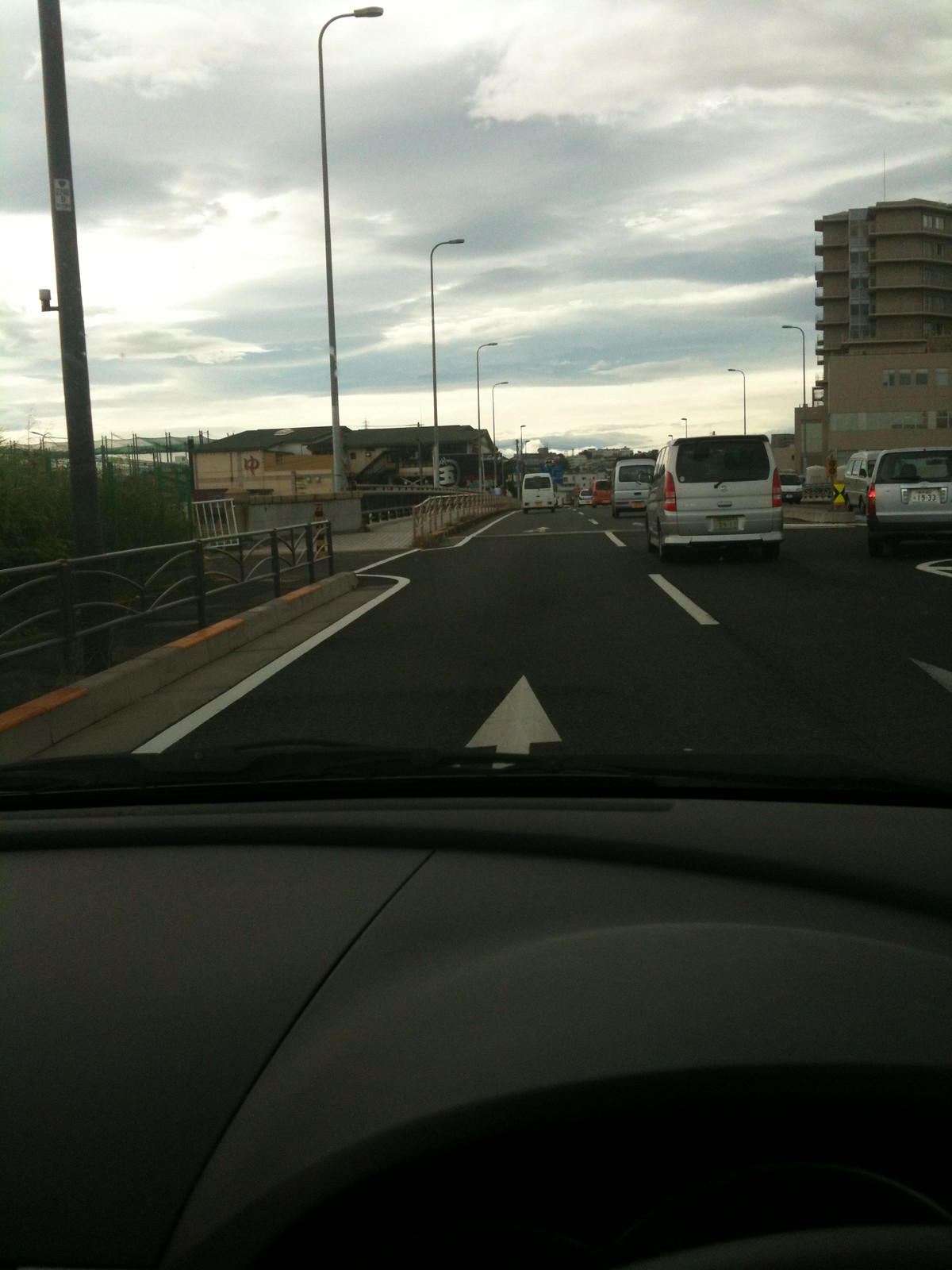The color photograph captures a scene viewed from behind the steering wheel, taken from the driver’s perspective on a foreign motorway or major road, seemingly during late afternoon or early evening as the sky shows heavy clouds with patches of blue. The dashboard, a dark gray, is partially visible along with the wiper blades. The driver is in the far left lane of a multi-lane road, possibly an interstate or highway passing through an urban area.

Ahead, a white minivan can be seen in the distance, while to the right, there are several cars including another white van, and a silver vehicle of similar design. Farther ahead on the right, a silver car is moving towards an on-ramp or off-ramp. There’s an array of colors among nearby vehicles including silver, black, white, yellow, and green.

To the right, the upper corner of a tall building, potentially a high-rise apartment with visible balconies suggesting it's residential, stands prominently. Along the sidewalk on the left, a railing separates the road from the pedestrian path. The sky appears overcast with heavy, possibly rain-laden clouds, adding to the atmospheric setting of the portrayed cityscape.